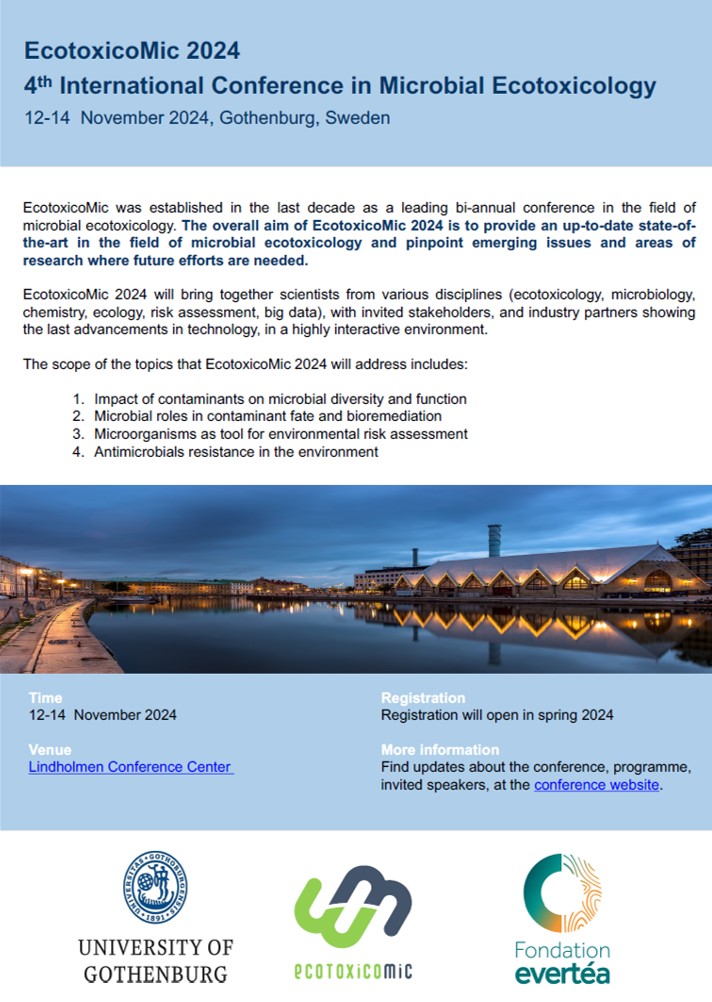The image is a detailed and organized color publication combining photography and graphic design, serving as an informational sheet for the "Ecotoxico MIC 2024," the Fourth International Conference in Microbial Ecotoxicology. The top section features a blue horizontal rectangle with darker blue text that reads, "Ecotoxico MIC 2024, Fourth International Conference in Microbial Ecotoxicology, 12-14 November 2024, Gothenburg, Sweden." Below this header, a white background with black lettering provides a brief description of the event, stating its aim to update the state-of-the-art in microbial ecotoxicology and highlight emerging research areas. The main portion showcases a horizontal photograph of the Lindholmen Conference Center, the conference venue, with a reflecting river on the left, a walking path, and surrounding architecture. This image is framed by a lighter blue rectangle that provides additional event details, including the dates, venue name, and registration information, which will open in spring 2024. The bottom part of the image, set against a white background, features the logos of the event organizers and sponsors: the University of Gothenburg on the left, "Ecotoxico MIC" in the center, and Foundation Everti on the right. The entire layout, approximately 6 inches high and 4 inches wide, combines elements of color photography realism and graphic design to effectively convey comprehensive information about the conference.